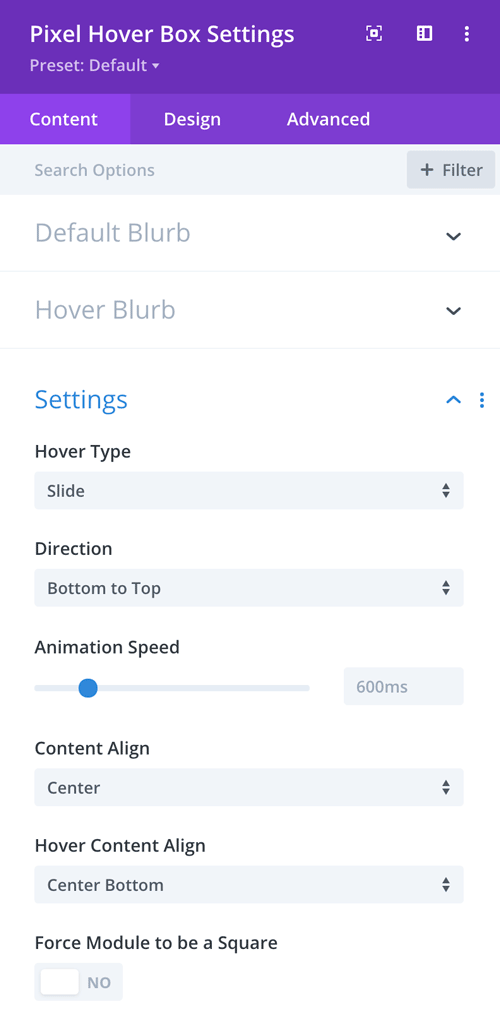This screenshot captures a segment of a mobile app's settings interface, specifically within the "Pixel Hover Box Settings" section. At the top of the screen, a purple rectangular header prominently displays the title "Pixel Hover Box Settings" in white font. To its right, a cluster of small white icons, whose specific functions are unclear, adds to the interface's design.

Directly beneath the header, in a lighter white font, the text "Preset: Default" is displayed alongside a downward-facing arrow, suggesting an expandable menu. Following this, a lighter purple bar includes a series of segmented options: "Content" is highlighted, indicating it is the currently selected tab, while "Design" and "Advanced" follow.

Below the tab options, a gray search filter bar contains the instruction "Search Options" and a button labeled "+ Filter" in lighter gray font.

Further down, the interface lists several settings in gray font, starting with "Default Blurb," which includes a black downward-facing arrow to the right. This is mirrored with the "Hover Blurb" option, also paired with a black downward-facing arrow.

Next, a section labeled "Settings" in blue font features a corresponding blue upward-facing arrow. Under this is the "Hover Type" setting in black font, followed by a light gray rectangular input area labeled "Slide" in black font, which includes an up-down arrow selector on its right side. The final item in the screenshot is the "Direction" setting, indicated in black font.

Overall, the settings interface is designed with a structured and layered appearance, using a combination of color-coded fonts and interactive elements to organize multiple options clearly and efficiently.